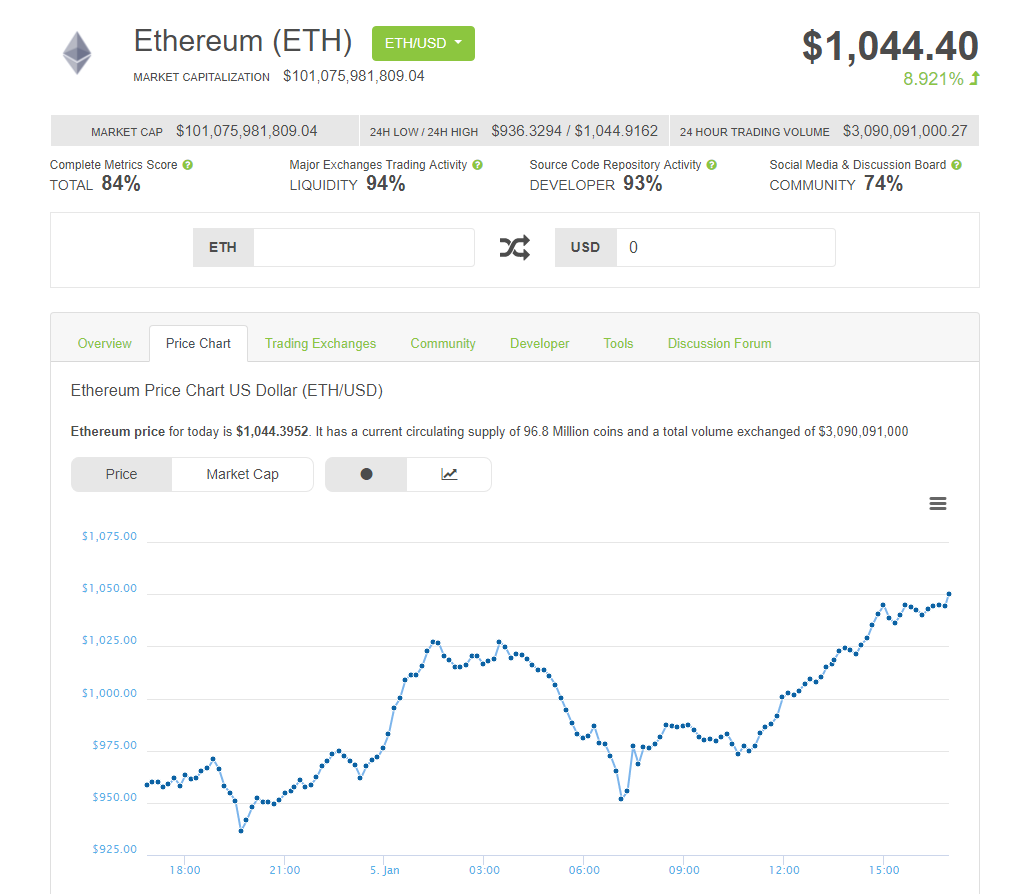This screenshot provides a comprehensive overview of Ethereum (ETH) data from a financial website or app. In the top-left corner, there's a gray, diamond-shaped logo, adjacent to the text "Ethereum (ETH)." Right next to it is a prominent green button labeled "ETH/USD" with a drop-down arrow.

Below this section, the market capitalization is listed as $101,075,981,809.04. On the right-hand side, a large bold dollar amount displays the current price of Ethereum: $1,044.40. Directly beneath this amount, in smaller green text, is an increase indicator showing "+8.91%" along with an upward arrow.

The following section includes multiple tabs showing key metrics: "Market Cap," "24 Low," "24 High," and "24H Trading Volume." Further down, there's another row detailing "Complete Metric Score," "Major Exchanges Trading Activity," "Source Code Repository Activity," and "Social Media and Discussion Board."

A conversion tool is also featured prominently, allowing users to convert between ETH and USD. At the bottom, various tabs are available for navigation: "Overview," "Price Chart," "Trading Exchanges," "Community," "Developer Tools," and "Discussion Forum," with the "Price Chart" tab currently selected. The displayed line graph illustrates the recent price trend for Ethereum.